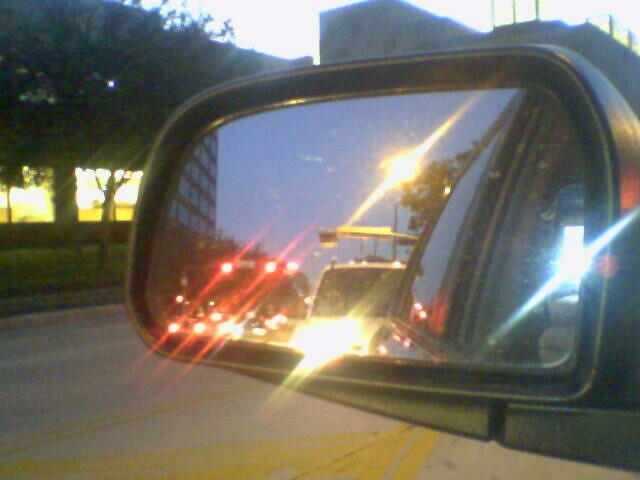This photograph, taken with a phone using flash from the driver's side mirror of a vehicle, captures a reflective nighttime urban scene. The primary focus is the car's side mirror, framed with black trim, revealing a view of various elements behind the vehicle. The reflection shows a white van immediately behind the car, illuminated by its lights, as well as other vehicles with their headlights on. The darkening sky is punctuated by streaks of light from street lamps and traffic lights, among which the overhanging stoplight stands out, glowing red. The image also includes blurred lines from the white, yellow, and red lights of other vehicles, street signs, buildings, and city infrastructure, creating a bright, hazy effect. Additional details include the roadway visible below the mirror, as well as some trees, grass, and sidewalks, emphasizing the city setting. The photographer’s hand holding the phone, with three fingers visible, and the glare of the flash are also reflected in the mirror, adding to the blurred texture of the image.